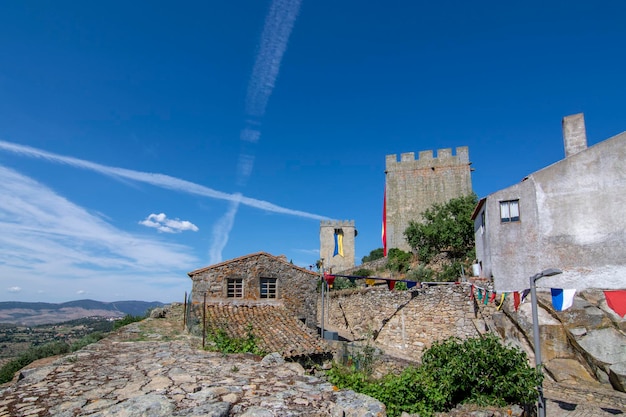This is a detailed color photograph taken outdoors during the daytime, showcasing a historic stone building, possibly a fort, situated atop a mountain or hill. The stone structure, built from numerous gray and brown blocks, features multiple components including a tall stone tower with a chimney and a smaller turret, reminiscent of a castle. The foreground is dominated by a stone walkway starting from the bottom left and extending towards the center, interspersed with typical rocky terrain and bordered by green vegetation on the right.

The background reveals gray mountains and a vividly blue sky with streaks of white clouds and visible contrails forming X and T shapes. Along the right side of the photograph, colorful pennant banners in red, white, blue, and green hang from a string attached to one of the stone buildings, adding a splash of color to the scene. The stone building itself features two forward-facing windows, and the scene is framed with calm mountain trails and puffy clouds, capturing the serene and historical essence of the location.